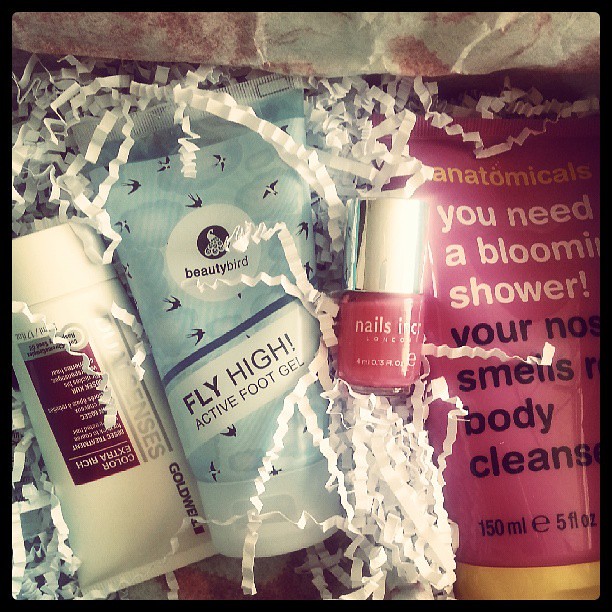The image showcases the contents of a beauty skincare gift box, filled with crinkled white paper for added presentation. On the left side, there is a white tube with a white cap labeled "Color Extra Rich," most likely a cream. In the center, there is a light blue squeeze bottle with a white cap and an image of flying birds. This bottle reads "Fly High Active Foot Gel" and is branded Beauty Bird. To the right of the foot gel, there's a smaller glass bottle of red nail polish with a silver cap. Further right, there's a large red tube with a gold cap reading "You Need a Bloomin' Shower. Your Nose Smells Body Cleanse." All these items are nestled within the decorative white shredded confetti, making it a visually appealing gift box of assorted beauty products.